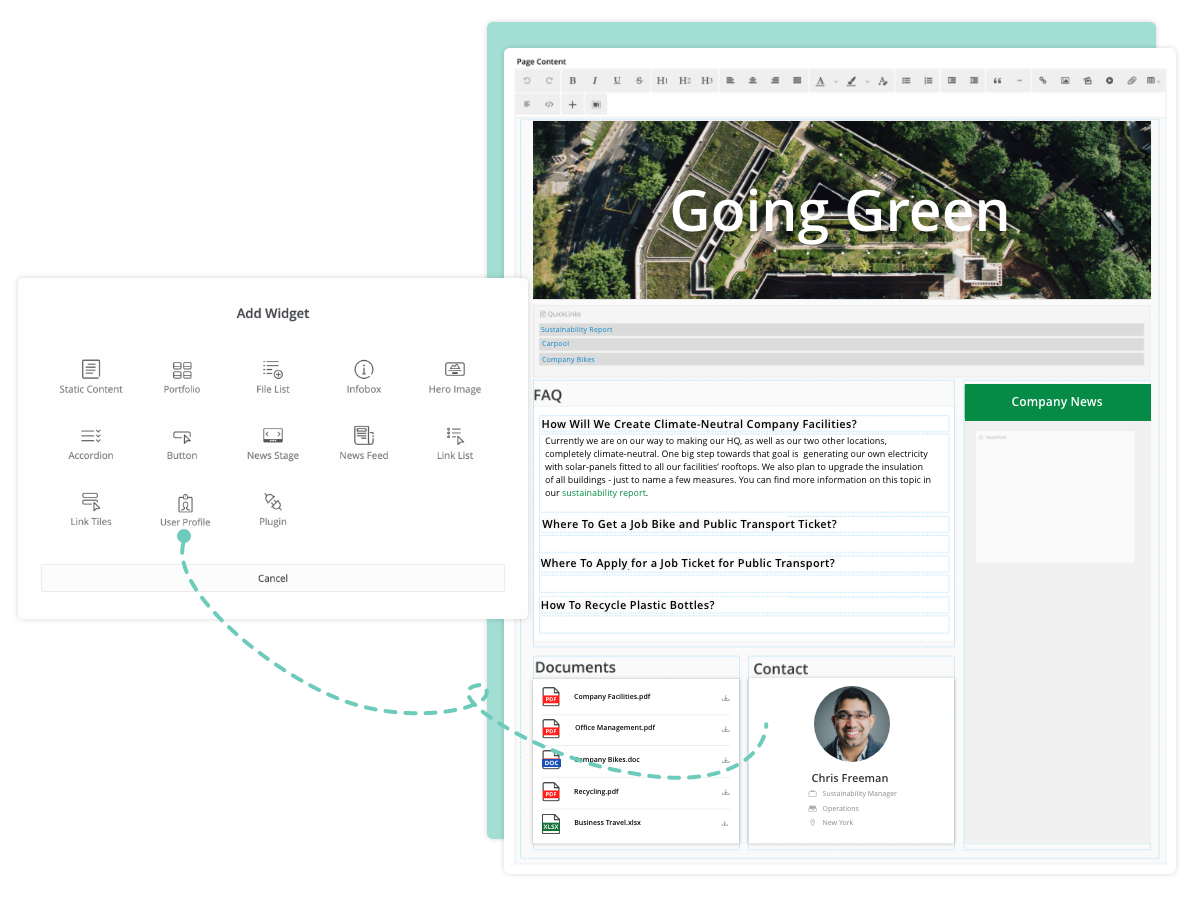This screenshot appears to be taken from a desktop publishing or web editing application, showcasing a workspace with a green background. In the center is a large white drafting area. 

At the top left corner, the bold black text reads "Page Content." Directly below are about 20 gray icons related to page formatting, arranged horizontally. These icons include options for Header 1, Header 2, justification tabs, font, font color, font style, image insertion, and more.

Within the central white area, there's an overhead view photograph of a lush, landscaped garden, prominently featuring the text "Going Green" in white across the center. Directly beneath this photo are three horizontal gray lines. To the left, in blue, are the headings: "Sustainability Report," "Carpool," and "Company Bikes." Below this, the bold black text "FAQ" is followed by another black heading: "How will we create climate-neutral company facilities." Here, a paragraph of information concludes with a blue hyperlink labeled "Sustainability Report."

Further down, three sections are separated by bold black labels: "How to Get a Job," "Bike and Public Transportation Ticket," and "Where to Apply for a Job Ticket for Public Transportation and How to Recycle Plastic Bottles."

At the bottom, there are two white squares. The left square, labeled "Documents," lists various document formats represented by icons of pieces of paper with red, blue, or green banners at the bottom. The right square, against a white background, features a "Contact" section in black text. It includes a circular image of a young man with short black hair and glasses, identified as "Chris Freeman" in bold black text.

A blue-green dotted line extends from Chris Freeman's image upwards towards the left, connecting to a pop-up window on the left-hand side of the screen. The pop-up window, titled "Add Widget" in black, displays three rows of different widgets available for adding to the page, indicating that this application is likely a web editor. The dotted line ends with a large blue circle under the widget labeled "User Profile."